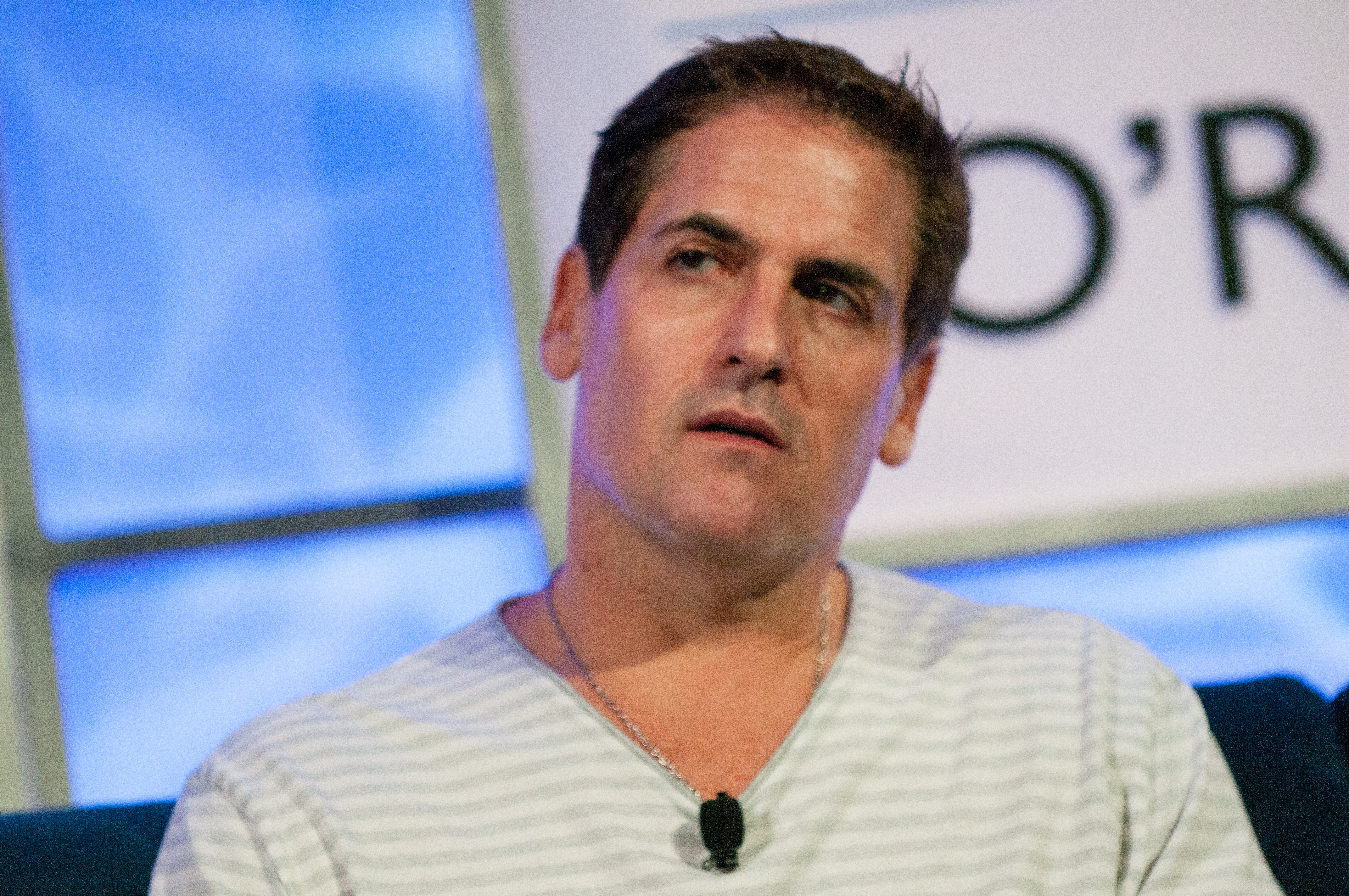In this image, we see Mark Cuban, seated indoors, likely in a studio or interview setting. The background is illuminated with light blue and white hues, possibly from a digital screen or window, adding a bright and lighted atmosphere. Centrally positioned, Mark has short brown hair and a square jaw, and he is wearing a white and gray striped V-neck long-sleeve shirt with a small black microphone clipped on it. His head is tilted upward as if he is listening intently but with a hint of skepticism, his mouth slightly open as if saying "huh." Around his neck is a white gold chain necklace. He is sitting on a dark navy blue couch. The upper right corner of the image features a partially visible white sign with black lettering, reading "O'R," though the complete text is cut off. The scene appears to be during an indoor interview, creating a professional yet engaging environment.